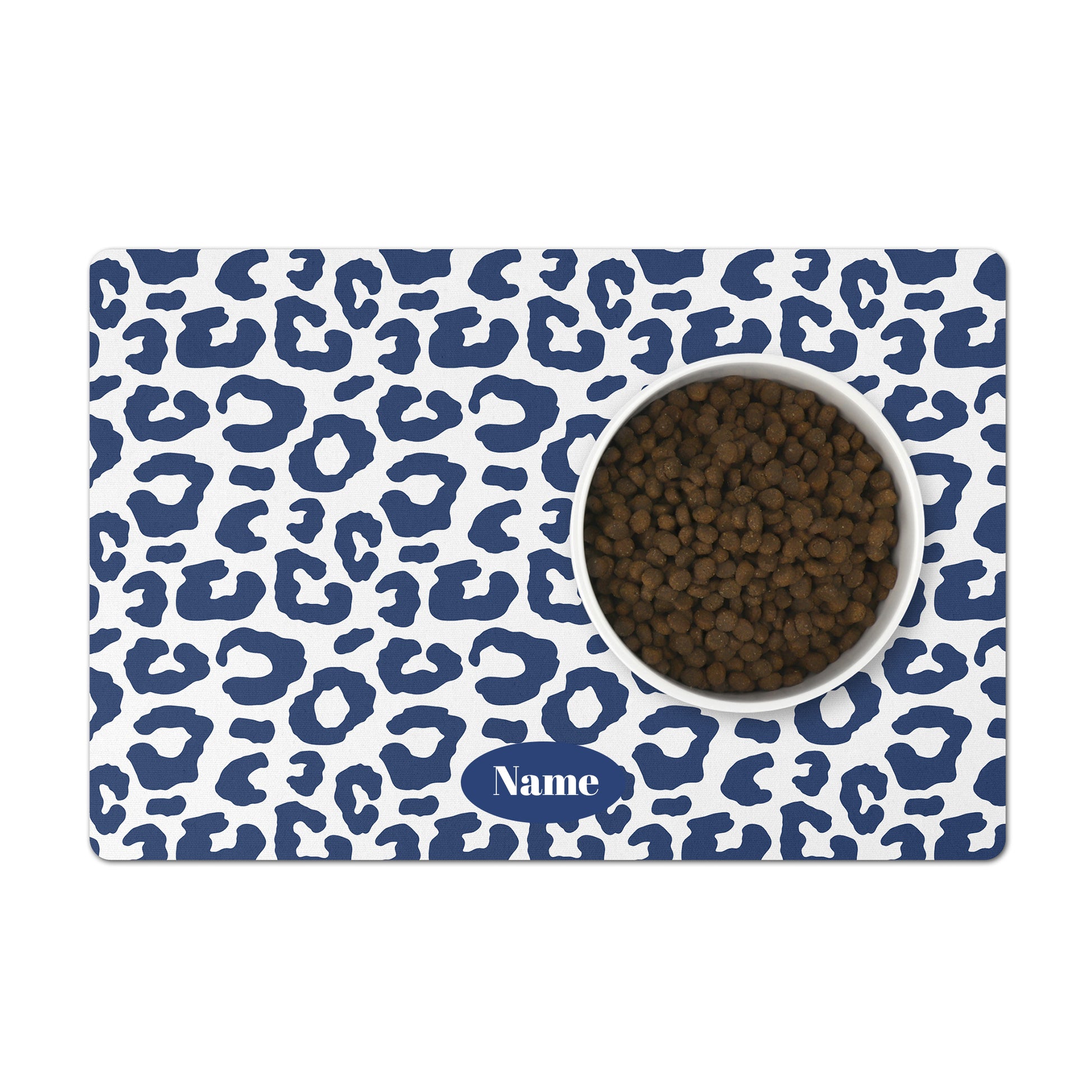The image features an overhead view of a white bowl situated on a blue and white leopard print placemat. The bowl contains small, round, dark brown pellets, which resemble dog kibble. Each piece of kibble is consistent in shape and size, with some exhibiting lighter brown hues. The background placemat displays a mix of full-leopard print circles and partial "C" shaped leopard spots, exclusively in blue and white shades. Positioned at the bottom center of the mat is a blue oval with the word "NAME" written in white, using a capital 'N' and lowercase 'a', 'm', 'e'. The scene is well-lit, offering clear visibility of all elements in the image.